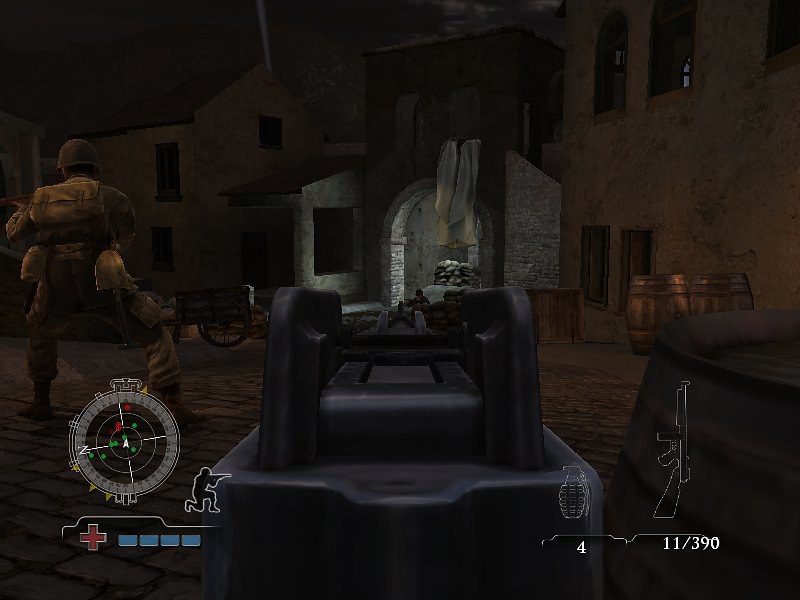In a nocturnal scene from a video game, a lone soldier patrols a stone-constructed courtyard, his rifle at the ready. Clad in a full uniform with additional weapons draped over his shoulders, he cuts a solitary figure under the dim light. His protective hard helmet completes his battle-ready appearance. In the background, wine barrels are scattered across the courtyard, offering a sense of the surrounding environment. A mysterious black object, possibly a cannon launcher, also stands out. Overlaying the image are computer-generated elements, including a compass and icons depicting a man on his knees holding a gun, a grenade, and a long-barreled firearm, adding to the immersive battle atmosphere of the scene.